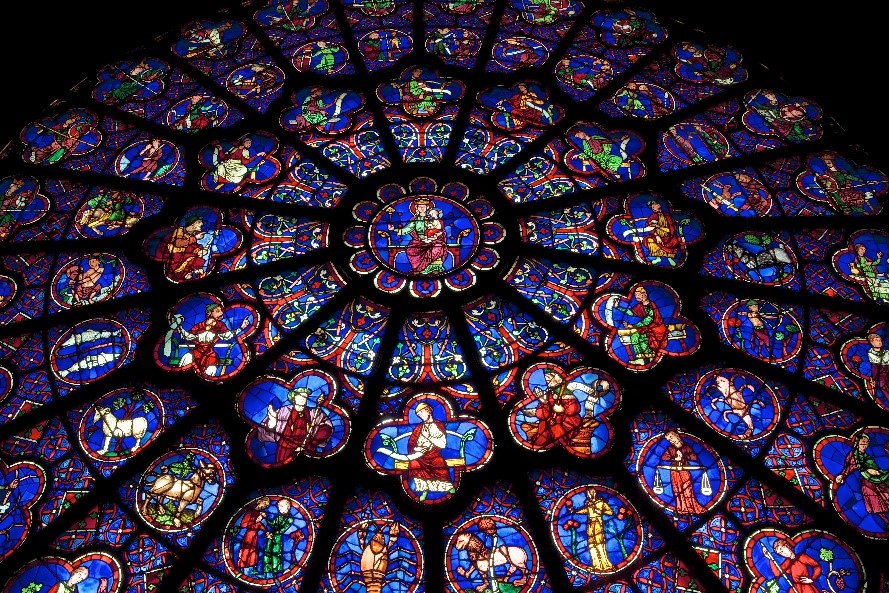The image captures the intricate stained glass ceiling of a cathedral, viewed from an indoor setting. At the center of this circular composition is a prominent stained glass depiction of a woman, perhaps a queen, holding a baby, reminiscent of a throne scene. Surrounding this central image are concentric rings of stained glass, each ring radiating outward like the spokes of a wheel. These rings are filled with vibrant and detailed scenes. Immediately around the central image, simpler designs fill the spaces. Beyond these, cloverleaf-shaped sections feature colorful depictions of various people, showcasing bright hues of blue, red, green, and yellow. Further outward, another ring includes images of both people and animals—such as a lobster-like creature, fish, goats, and horses. The entire ensemble is held together by a black radial frame, creating a spiderweb effect. The image is viewed diagonally, with the bottom part appearing larger and the upper corners revealing the black background. The vivid colors and detailed craftsmanship of the stained glass make the ceiling a breathtaking focal point.